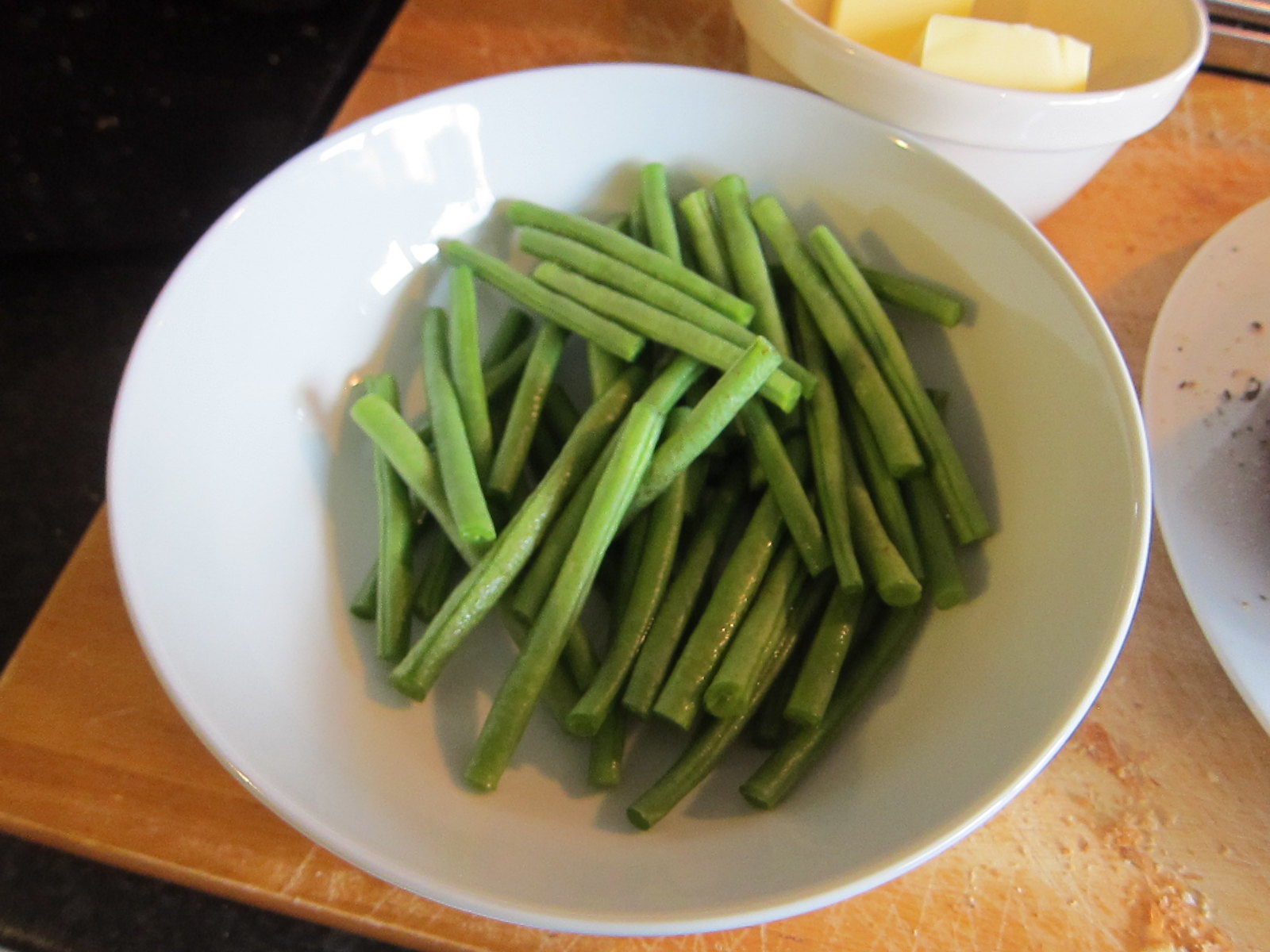This indoor color photograph captures a detailed scene centered around a round, off-white ceramic bowl filled with approximately 40 to 50 cut green beans. The green beans, meticulously arranged in a vertical fashion, are of a uniform length of 4 to 5 inches, with their ends and tips trimmed. The elegant, shallow bowl sits on a wooden table that resembles a cutting board, evidenced by visible knife marks and scattered crumbs. Above the bowl with the green beans, a higher bowl with a rim, potentially containing two sticks of butter, can be seen. To the right of the central bowl, there is a partial view of a white ceramic plate with a few black crumbs on its surface. The green beans appear uncooked and the entire setup is captured in sharp focus under good lighting, highlighting the textural details of the beans and the rustic surface of the wooden table.